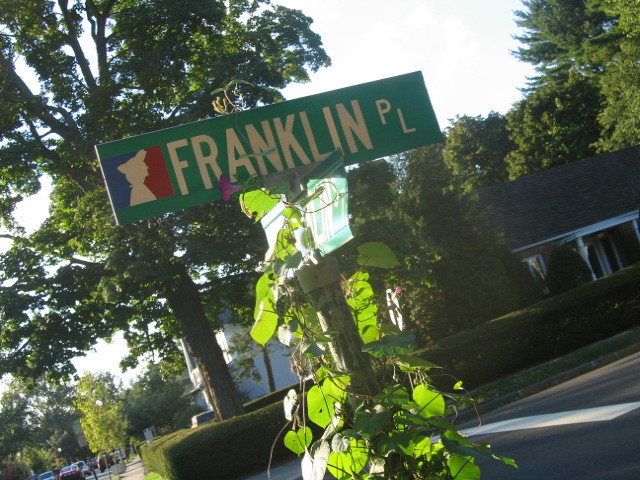This image captures a green rectangular street sign with white lettering that reads "Franklin Pl," signifying Franklin Place. To the left of the text, there is a blue, white, and red silhouette of a Revolutionary-era soldier in profile. Below this, another street sign faces the opposite direction, though the name is obscured by sun glare. Both signs are mounted on a metal post with a flat top, partially covered by cascading green ivy. In the background, across the street, a charming house with a mansard roof and a neatly trimmed row of hedges completes the picturesque scene.